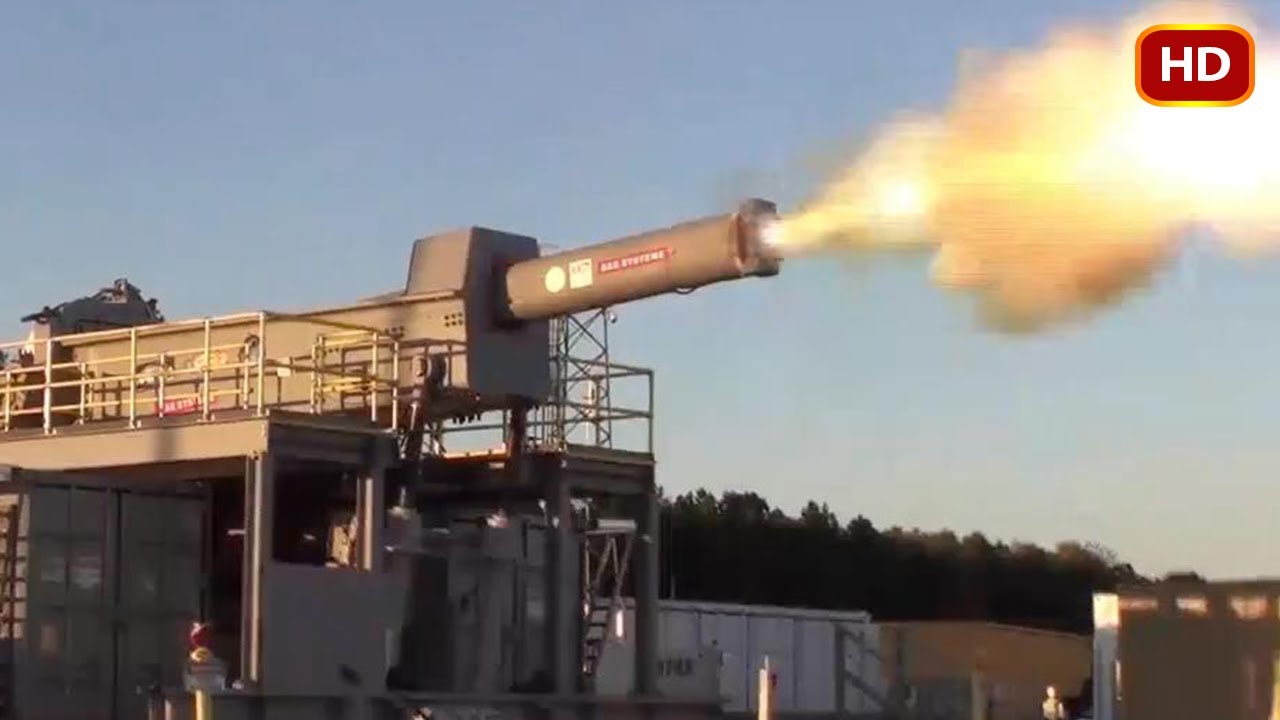The image captures a modern, industrial-looking cannon, possibly in a testing facility, mid-firing. The cannon, which deviates from traditional wartime designs, is securely mounted on a robust metal scaffolding structure. It has several tubes protruding from its sides and appears to expel hot gases and a bright cloud from its muzzle, indicative of a recent firing. Surrounding the cannon are various rails, steps, and ladders, emphasizing its elevated position. The background reveals the silhouette of trees and some indistinct industrial structures beneath a blue sky adorned with light clouds. The top right corner of the image features an "HD" label, highlighted in white, surrounded by a red frame with a gold border. The overall scene is devoid of people, focusing solely on the imposing, active cannon and its immediate surroundings.